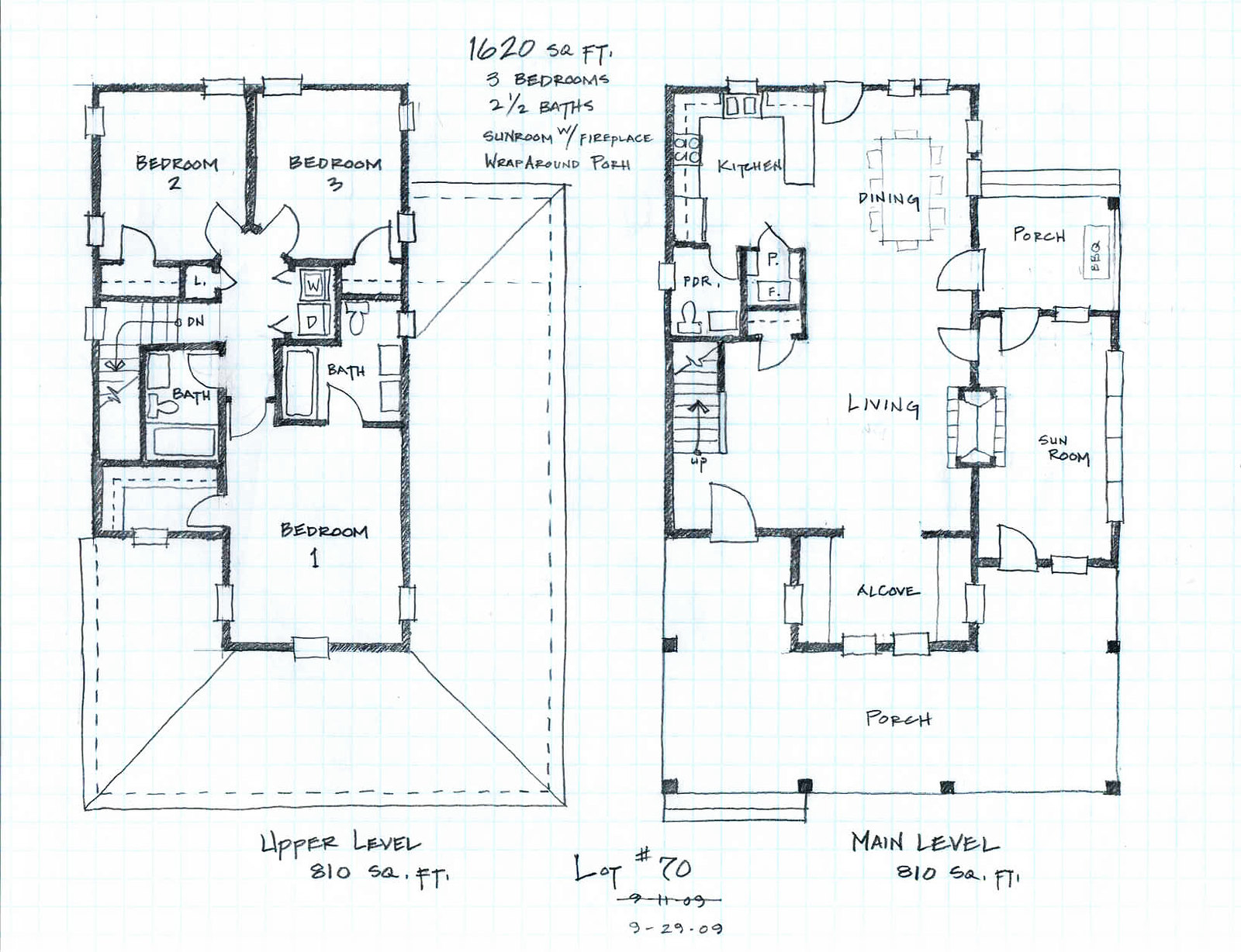This detailed blueprint sketch showcases the layout of a modern house. The left section illustrates the first floor, featuring Bedroom One, Bedroom Two, and Bedroom Three, along with spaces allocated for two bathrooms. The total area of the house is specified as 1,620 square feet, and it includes three bedrooms and two and a half bathrooms. On the right side, the blueprint details the communal living spaces, including a kitchen, dining room, and a living room, as well as an adjacent porch and a sunroom, complemented by an additional porch. The blueprint provides a comprehensive view of the house's design and layout.